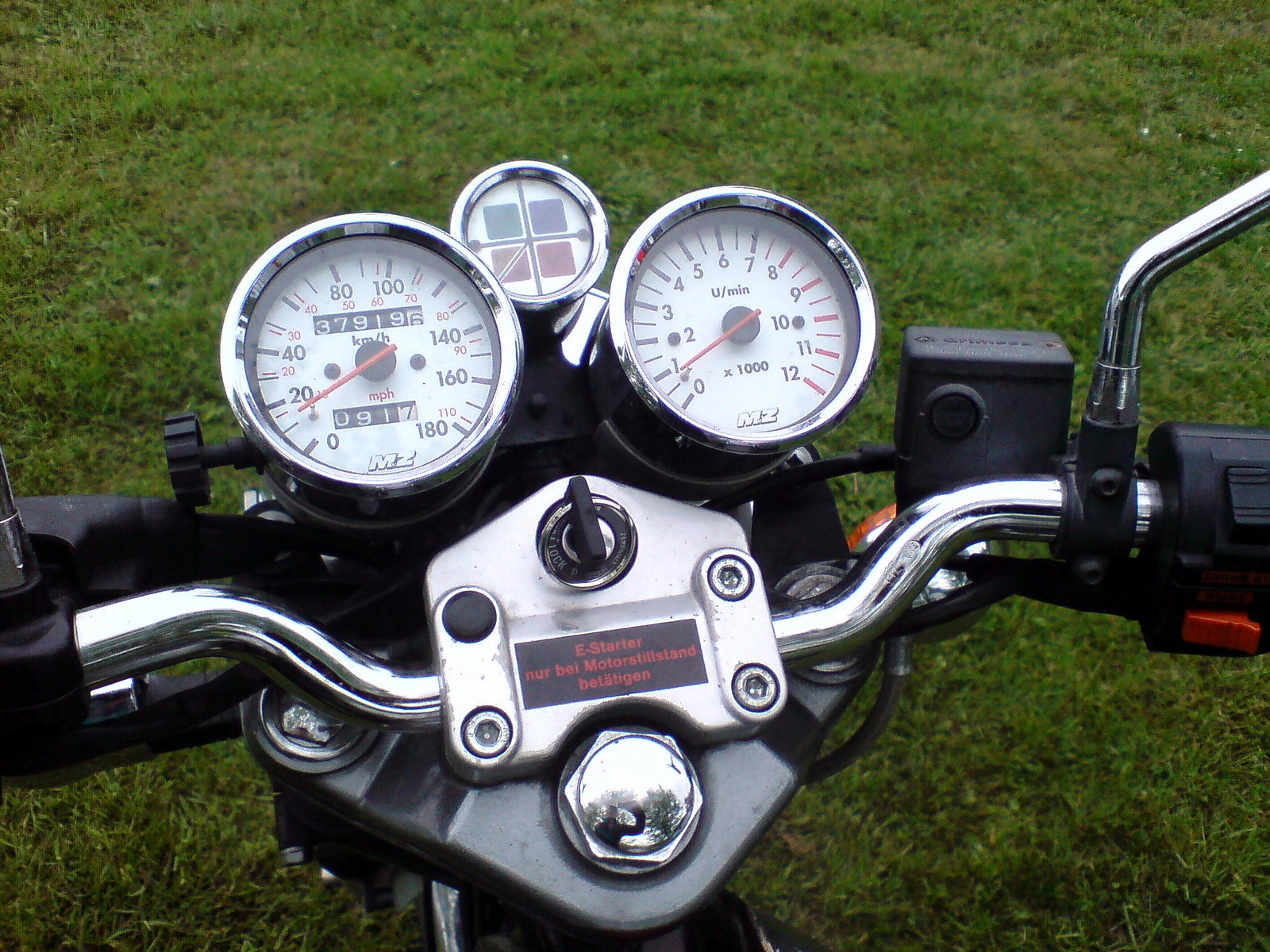This photograph, taken from the point of view of a motorcycle driver, captures a detailed view of the motorcycle's handlebar and instrument cluster. The handlebars themselves are partially visible, showing where the mirrors are mounted. The right mirror mount features a switch with red and black toggles. To the left of the left mirror mount, there is a small black box, likely a video camera. 

The instrument cluster boasts three prominent, chrome-trimmed, round gauges. The left gauge measures speed in kilometers per hour (KM/H), ranging from 0 to 180 in black, with an additional scale in red indicating 0 to 110 miles per hour (MPH). The odometer displays a reading of 37,919 with a small digit turning over from 6 to 7, while a secondary counter below shows 091 with a 7. The speedometer features a vivid red needle on a black dial.

The right gauge is a tachometer, marked as U/min x 1000, which likely stands for revolutions per minute (RPM) with a range from 0 to 12. At the bottom of both the speedometer and tachometer, the gauge is labeled with the letters "MZ." 

Above these two main gauges is a smaller, circular gauge displaying four color-coded sections: green, blue, and two red squares, the function of which is not specified. 

Below the main gauges, there is a small digital display featuring the German text "E-starter Nür Bei Moto Schild Stand," which roughly translates to "E-starter only in Moto shield stand." This area also includes what appears to be the ignition key.